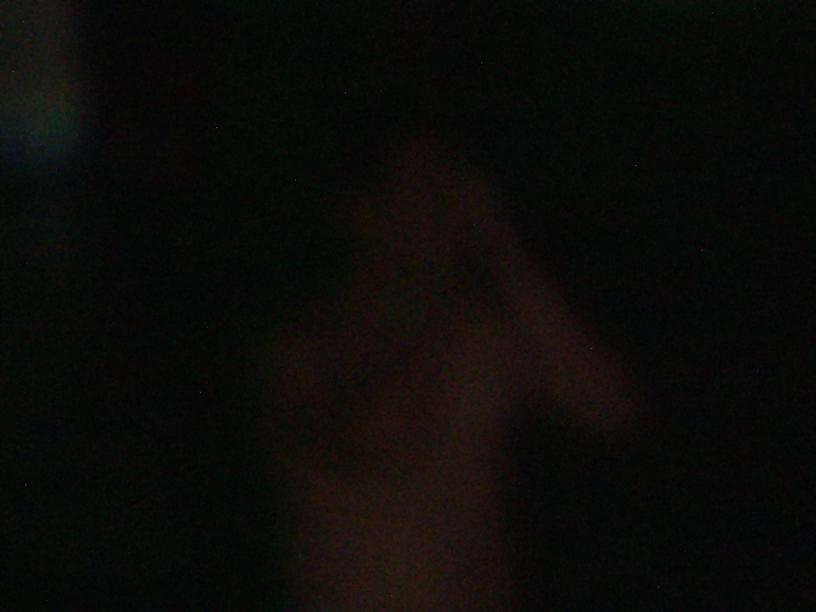The image is an extremely blurry, pitch-black nighttime photograph featuring a vague, barely discernible figure that appears to be a shirtless man. The man is positioned in the middle of the image with his arms raised, as though his hands are either obscuring his face or engaged in a rubbing motion, reminiscent of a crying pose. The top left corner of the photograph contains a smudge of white-blue or light green light, potentially resembling the outline of fire or an unclear shape. The figure in the photograph has short brown hair, and the overall scene is so indistinct that it creates an impression akin to viewing it without glasses or through an obscured lens.